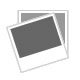The image showcases an assorted gift box containing multiple Shinola-branded items, meticulously arranged on a white surface. Dominating the center is a wristwatch featuring a brown leather strap with white stitching and a black dial that displays the time as 6:20. Placed alongside the watch on the left, is a black leather wallet with the embossed text "Shinola." Adjacent to these items are two small boxes: a black one, marked "Shinola Detroit Leather Care Balm," located in the top left corner, and a wooden box labeled "Shinola Leather," positioned in the top right corner.

Below these boxes, a pair of cards can be seen—a black card with "Shinola Detroit" in silver writing and a tan card inscribed with "Where America is Made," followed by a smaller, illegible paragraph of text. Additionally, a plain black square sheet of paper and another black card resembling a credit or debit card are also visible near these items. The overall composition highlights the craftsmanship and branding of Shinola products, emphasizing their Detroit origin and American-made quality.